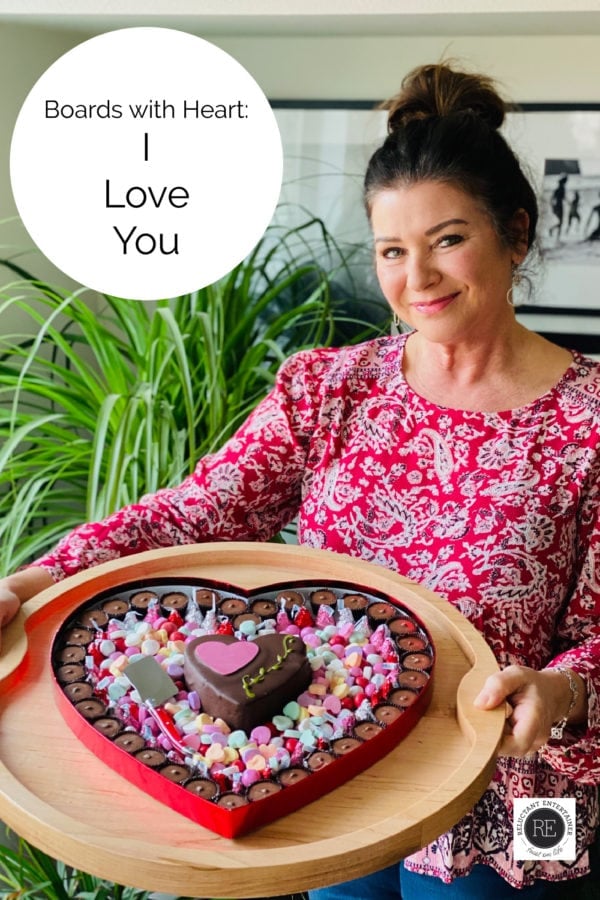In this image, a woman in her 40s or 50s, with dark brown hair styled in a ponytail, is smiling and slightly tilting her head. She is wearing a red blouse adorned with white and brown floral patterns, paired with blue jeans. The woman is holding a circular wooden tray that prominently features a heart-shaped container filled with various Valentine's Day-themed candies. The container includes small, round chocolates, colorful heart-shaped candies, and a larger heart-shaped chocolate or brownie in the center. Additionally, there are possibly some Hershey's Kisses scattered among the candies. In the top left corner of the image, a white circle contains the words "Burst With Heart, I Love You." Behind her, there is a green plant and a picture frame, adding to the warm and festive atmosphere of the scene.